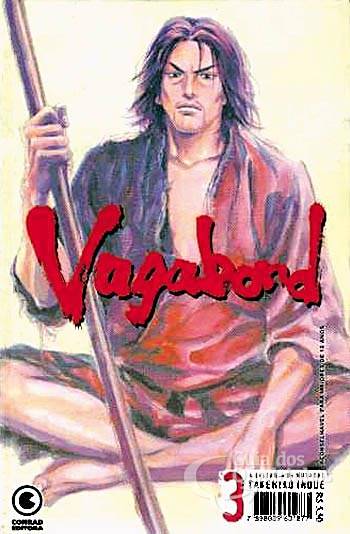The image is a cover that could belong to a comic or a novel, presenting a vividly detailed, full-color drawing of a male warrior. The warrior, a white male, sits cross-legged on the ground in an Indian style, his feet are bare. His long brown hair, accented with possible hints of purple, is parted in the middle and falls almost to his shoulders, fraying outwards. He holds a long, brown wooden staff in his right hand, pointed diagonally upward. His left hand rests on his left thigh. He is dressed in a traditional, loose-fitting robe characteristic of Japanese attire; the robe is predominantly red with a striking black section on his left shoulder, and it features a large middle opening that exposes his chest.

The background of the image is a subtle blend of yellow with touches of white, adding a warm tone to the scene. Centered around chest height on the warrior, the title "Vagabond" is displayed in stylized, red text, giving the cover a bold focal point. There's a distinctive logo resembling a pac-man shape in the bottom left corner, and the bottom right corner features a black barcode accompanied by a prominent red number three, likely part of a series indicator.